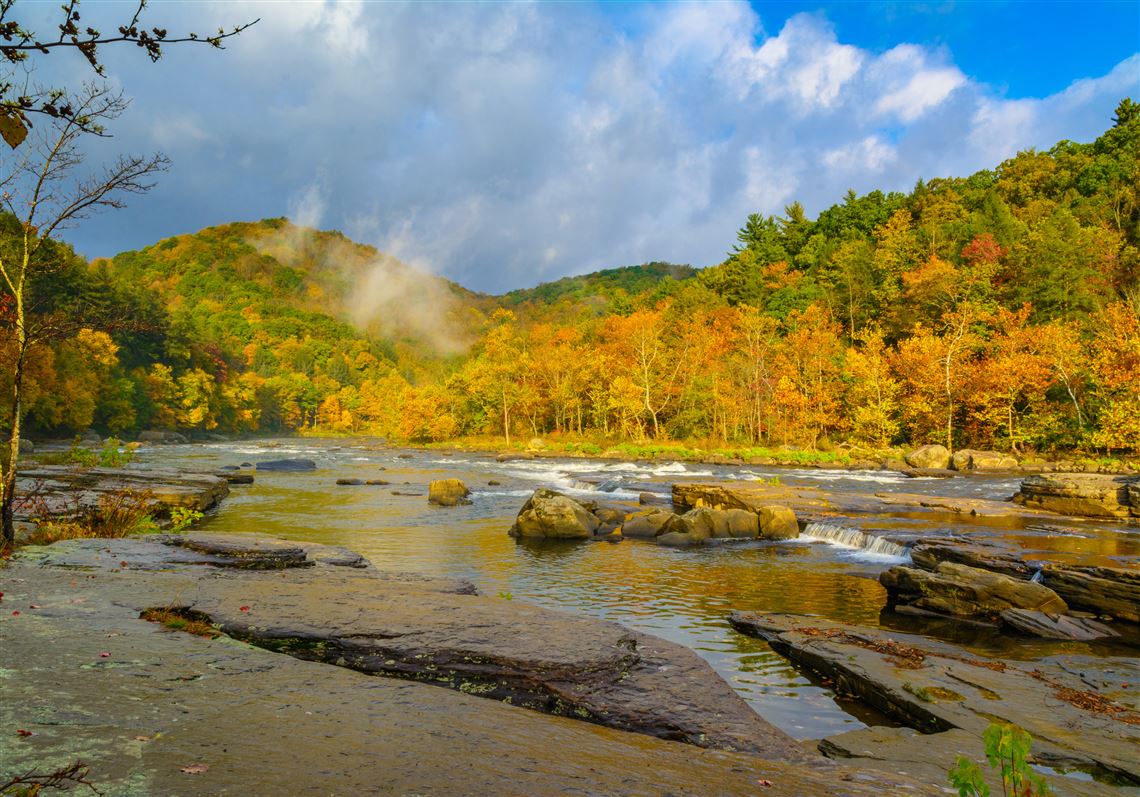This captivating photograph captures a serene wooded area in the midst of fall, characterized by rolling hills and a meandering stream. The stream displays a combination of calm sections and gentle rapids, where tiny white-capped waves break over rocks. Granite-like boulders are scattered throughout the waterway. The scenic banks are mostly flat and rocky, possibly shale, providing a smooth foreground for the viewer.

In the background, the hills are cloaked in a vibrant tapestry of trees exhibiting the spectacular colors of autumn. Varying shades of yellow, gold, and green dominate the foliage, with hints of red and orange adding to the colorful display. At the crest of the hills, the trees lean more towards green, transitioning to brighter hues as they reach the riverbank.

The sky above the landscape is a brilliant blue, interspersed with wispy clouds that enhance the overall beauty of the scene. This picturesque area, likely a perfect spot for camping, is accentuated by the presence of small waterfalls created by the different elevations of rocks along the stream. The harmonious blend of natural elements makes it a truly enchanting depiction of nature in fall.